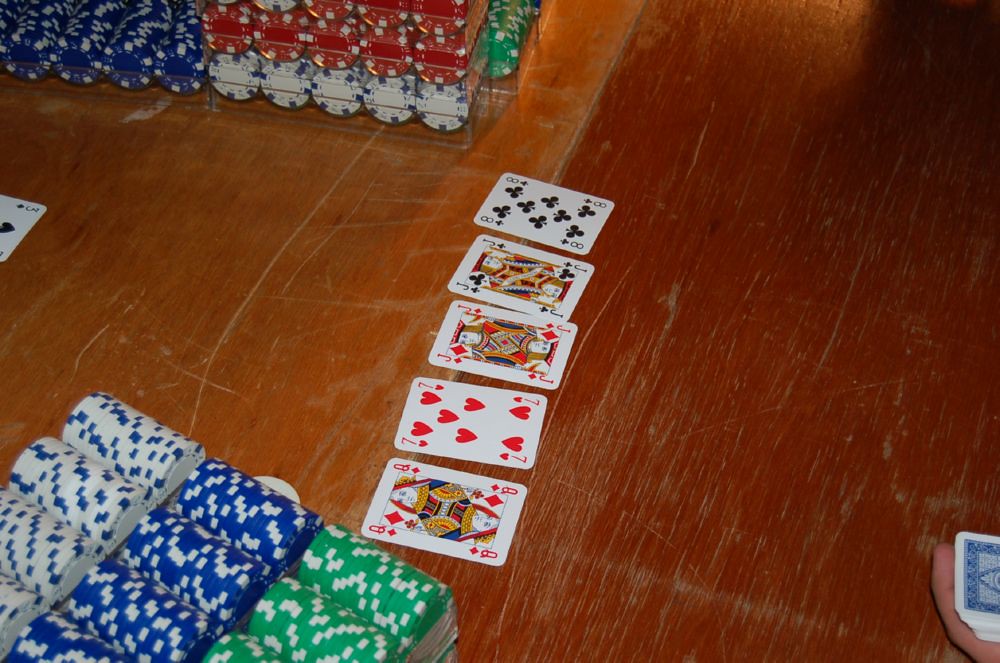The image depicts an intense poker game set on a well-worn, reddish-brown wooden surface covered in scratches. Scattered across the table are several playing cards: the Queen of Diamonds, Seven of Hearts, Jack of Diamonds, Jack of Clubs, and Eight of Clubs. In the top left and bottom left corners, a variety of poker chips are visible, including blue and white, red and white, predominantly white with blue accents, and green chips with additional accents. Near the left side of the table, a partially visible Three of Spades card sits in the frame. The bottom right corner reveals a player's hand, where they are holding a set of cards. The backs of these cards display a white border with a classic blue pattern. Lastly, the top right corner features a shadow, partially obscuring the light source and adding a touch of mystery to the scene.